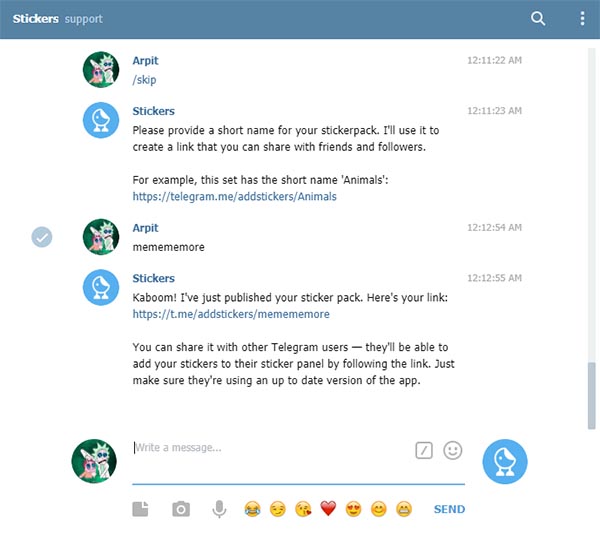The image is a slightly rectangular screenshot capturing a conversation between a user (RPIT) and an AI assistant named Stickers on a messaging platform. At the top, a grayish-blue horizontal banner contains the elements: "Stickers" in bold on the left, followed by the word "Support" in regular font, with a search icon and a three vertical dots icon appearing on the right side.

Below the banner, the conversation unfolds on a white background, with each participant represented by their respective avatars. The user, RPIT, initiates the conversation by typing "/skip." Stickers replies, asking the user to provide a short name for their sticker pack, explaining that this name will be used to create a shareable link. An example link structure is provided: "https://telegram.me/addstickers/animals."

RPIT responds with "name: me more." Stickers confirms the creation of the sticker pack with the enthusiastic message, "Kaboom, I've just published your sticker pack, here's your link: https://t.me/addstickers/mememore. You can share it with other Telegram users, who will be able to add your stickers to their sticker panel by following the link. Just make sure they're using an up-to-date version of the app."